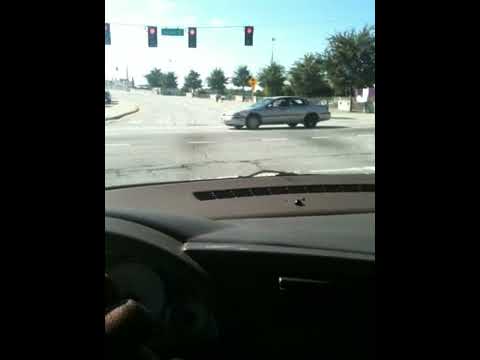This image captures the view from inside a car, likely taken by the driver, looking out through the windshield. The black dashboard and partial instrument panel are visible in the foreground. Outside, the scene reveals a gray road where a silver sedan is crossing from the left, as the car waits behind a set of four traffic lights, all glowing red. Suspended between the traffic lights is a green street sign with white lettering, although the text is unreadable. The background features a row of green trees against a clear blue sky with a patch of glare on the left side. This scene comprises the central panel of a triptych, with solid black borders making up the left and right panels.